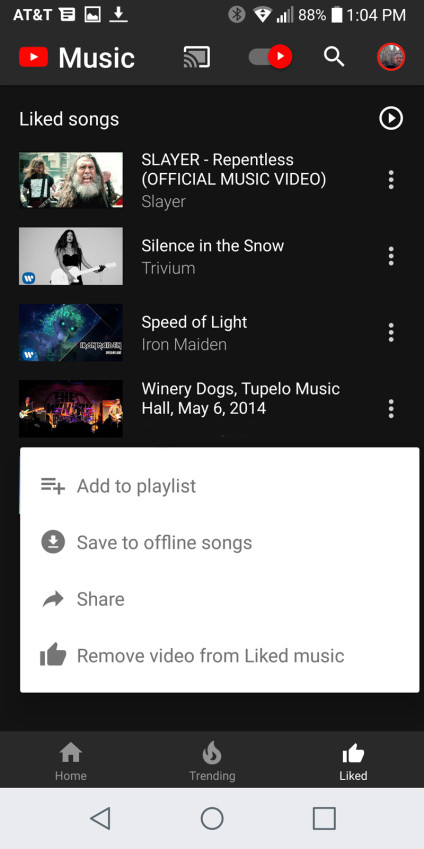A mobile screenshot of YouTube Music displaying a list of liked songs is shown on a predominantly black background. The top status bar indicates the screenshot was taken at 1:04 PM, with the phone's battery at 88%, and the network provider AT&T is visible on the upper left. Below this, the YouTube Music logo is clearly displayed. A red slider is positioned on the right side of the screen, and a profile picture with a red border is seen in the top right corner.

The main section reveals a list of liked songs in white text. The first song is "Repentless" by Slayer, featuring a thumbnail of a man with a gray beard, labeled as the official music video. The second song is "Silence in the Snow" by Trivium, with a thumbnail showing a woman playing a white guitar against a gray backdrop. The third is "Speed of Light" by Iron Maiden, accompanied by a thumbnail of a blue-grayish alien creature with greenish hair. The final song displayed is "Tupelo Music Hall, May 6, 2014" by Winery Dogs, with a thumbnail depicting the band performing.

At the bottom of the screen, a white text box provides options such as "Add to Playlist," "Save to Offline Songs," "Share," and "Remove Video from Liked Music."